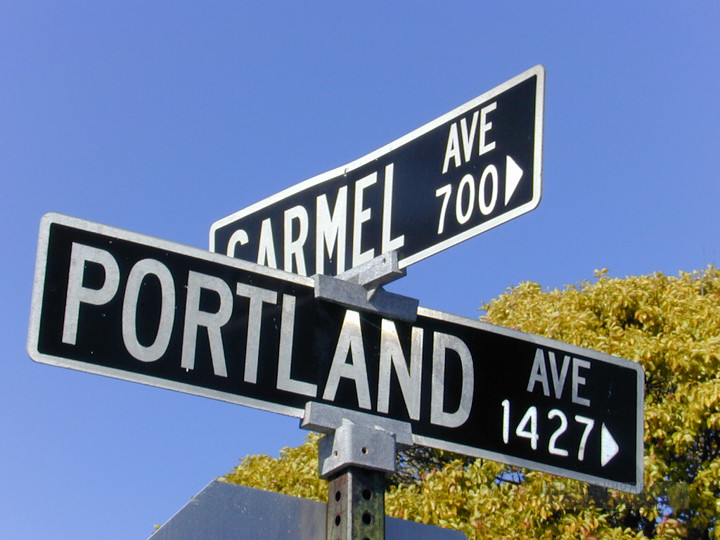This is a rectangular, close-up photograph capturing two intersecting street signs at an intersection, set against a vibrant blue, cloudless sky. The signs are mounted on a square, perforated metal pole with round holes visible on the front and side. The top sign is outlined in white with a black base and features white writing that reads "Carmel Avenue 700," with an arrow pointing to the right. Below it, the second sign shares the same black and white color scheme and reads "Portland Avenue 1427," with an arrow pointing downward. The intersection of these two signs creates a crisscross pattern. In the background, a yellow tree or large bush rises into the frame from the bottom right-hand corner, adding a touch of nature to the urban scene. Another sign appears to be attached to the pole but is facing away from the photographer.